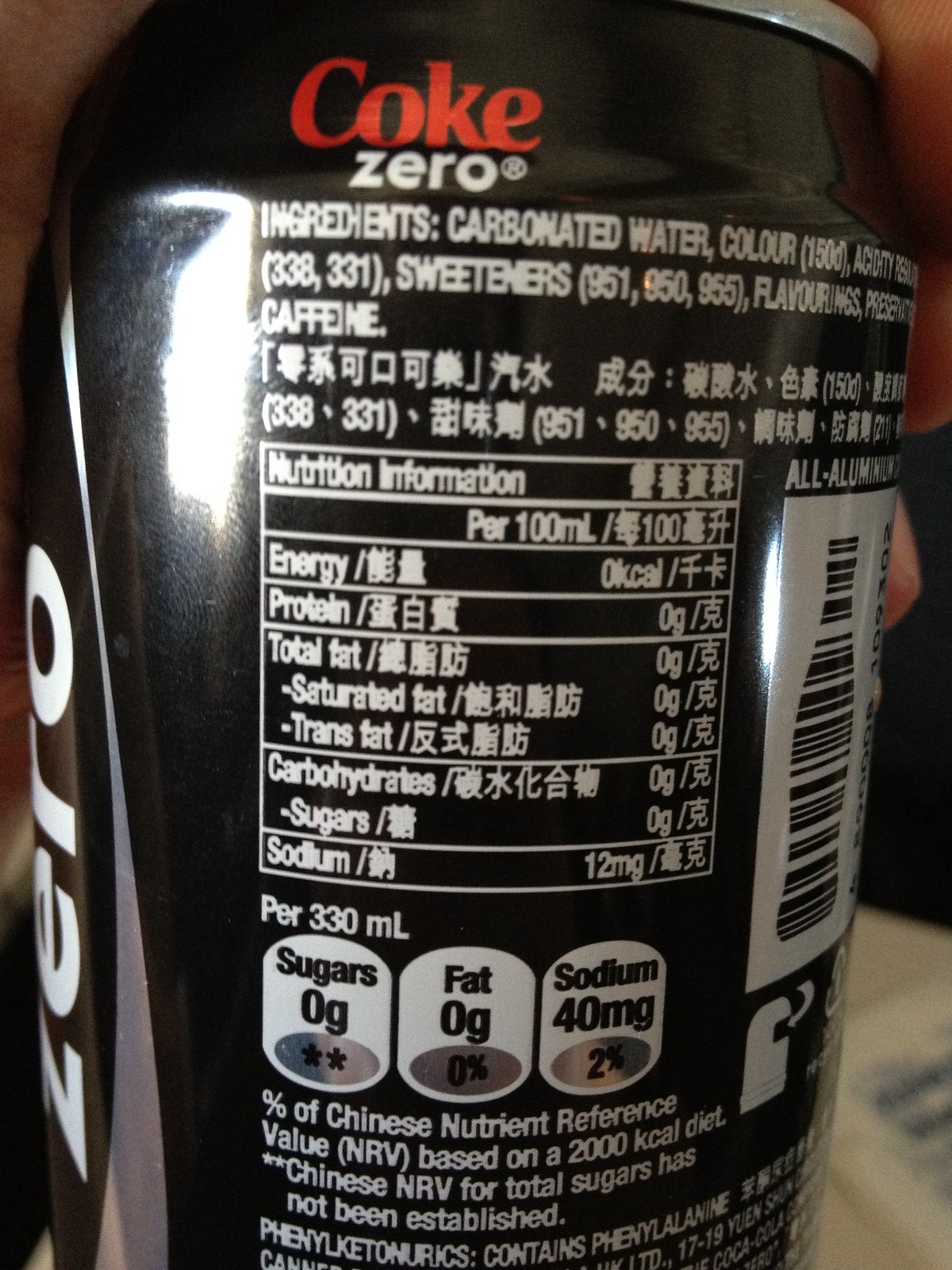This detailed color close-up photograph captures the back of a 12-ounce Coke Zero can, prominently featuring its black labeling with silver and white text. The can’s design includes red text spelling "Coke" and white text for "Zero," along with a distinctive grey stripe that runs vertically, and "Zero" written vertically in white along the left side of the can. The top band around the lid is silver.

Central to the image is a block of nutrition information written in both English and an Asian language, possibly Japanese or Chinese. This block is clearly legible, revealing details such as sugar content of 0 grams, fat content of 0 grams, and sodium content of 40 milligrams. Below this, additional nutritional references in Asian characters can be seen, indicating elements like energy, protein, and total fat, all listed as zero.

The photo also contains minor elements like a barcode designed to look like a bottle on the far right, and a light glare on the left side of the can. Partial fingers holding the can are visible in the upper right of the frame, indicating that the can is being held up for the photo. The overall image is clear and in good focus, with a white object faintly visible in the lower right background.